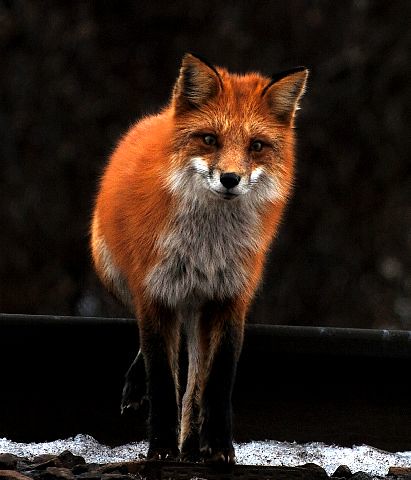In this photograph, a striking orange-red fox stands out vividly against a black background, likely taken at night. The fox, holding the camera's gaze with its intense eyes, has prominent white fur around its mouth that extends down to its chest. Its fur is predominantly an enchanting mix of orangish-red and rusty brown, with darker, black-tipped legs, and a black-tipped tail visible behind it. The fox’s nose and whiskers are particularly dark, creating a sharp contrast with its lighter fur. The ground beneath the fox appears rocky and icy, suggesting a cold environment, possibly winter, with some snow visible. The backdrop is quite blurred, making it hard to discern specific elements other than a curb or elevated platform behind the fox, from which it may have stepped down. Amidst the darkness, the absence of foliage, plants, or any other life suggests the fox is alone in this stark, wintry scene. The image is devoid of timestamp or text, allowing the natural majesty of the fox to command full attention.